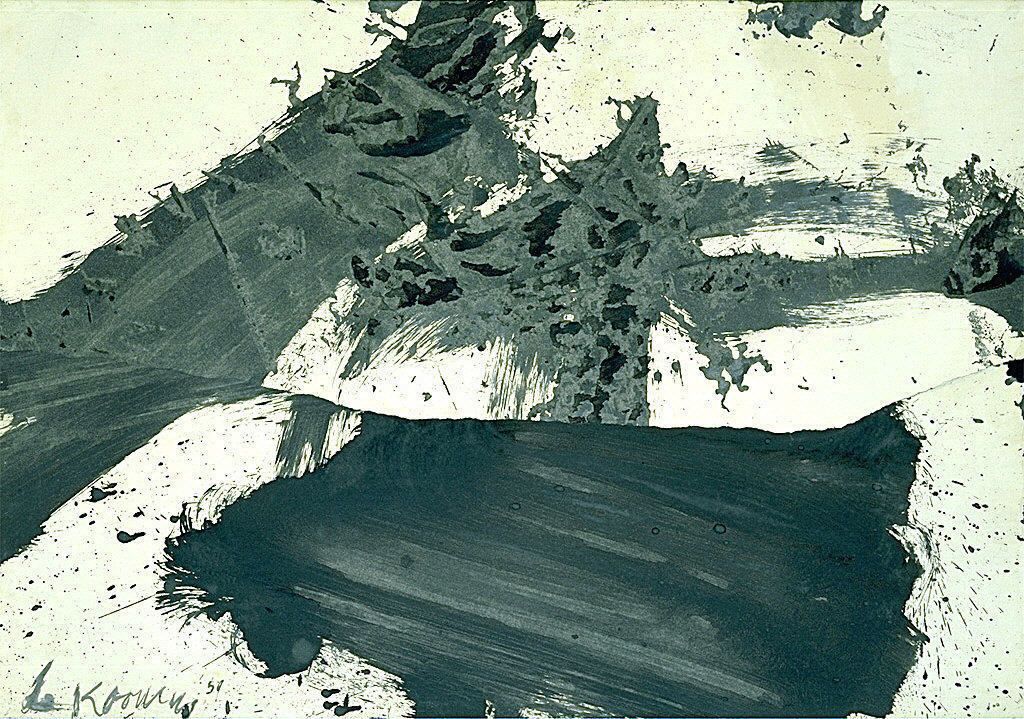This is an abstract piece of modern art, presenting a visually intriguing composition primarily in black, white, and various shades of gray. The painting's background is an off-white canvas, appearing slightly more beige and splotchy towards the top. Scrawled in cursive in the bottom left corner is a signature that is difficult to decipher but appears to include the initials "L" and "K." 

Throughout the composition are dynamic splashes and splotches of dark gray and lighter gray paint. Notable features include a large, dark gray almost black swatch towards the bottom, lighter gray splotches with darker details across the upper left and middle center, and numerous tiny dark gray spots that dapple the canvas sporadically. The paint appears to have been applied with broad, sweeping brush strokes and possibly even by hand or with a large tarp, creating an appearance of ink splatters. The random, otherworldly shapes and the absence of recognizable organic forms—such as plants, people, or buildings—contribute to the painting's deeply abstract nature. The visible brush strokes and erratic patterns suggest a spontaneous and energetic application process, enhancing the sense of abstract expressionism in the artwork.